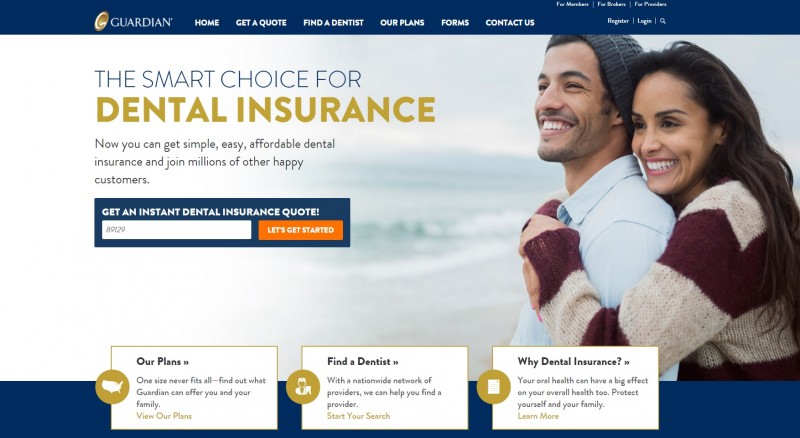This is a screenshot of a website featuring a dark blue navigation bar at the top. In the left corner of the bar, the website's name "Guardian" is displayed in white text, accompanied by a 3D orange circle logo. The navigation bar includes several buttons, labeled "Home," "Get a Quote," "Find a Dentist," "Our Plans," "Forms," and "Contact Us." On the far right of the bar, there are options to "Register" or "Log In."

Below the navigation bar is a photo depicting a cheerful scene by the ocean. A Latino woman and man stand close together, with the woman affectionately hugging the man. They both appear to be dressed for brisk weather. The woman, who has long, flowing brown hair and is smiling warmly, is wearing a beige sweater with black stripes. The man, also smiling, has brown hair partially covered by a beanie and is dressed in a blue button-up shirt. The backdrop of the ocean complements their joyful expression, highlighting a serene and pleasant moment.